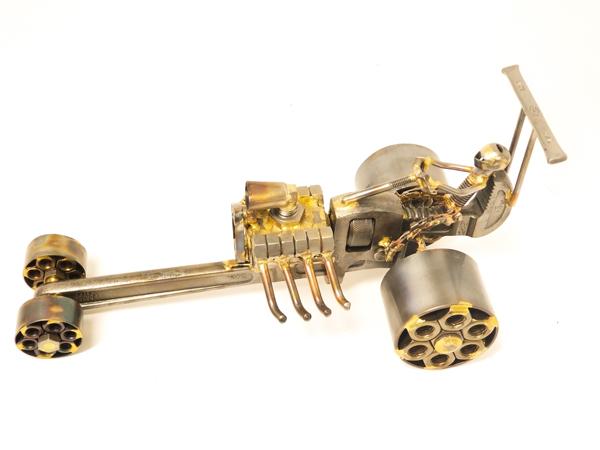The image is a horizontal photograph showcasing a detailed metal sculpture resembling a hot rod. The vehicle is constructed from various repurposed metal tools and parts. The base frame is made from an extended wrench, with the vice part serving as the seat for a small driver figure that looks like a metallic space alien. The rear of the vehicle features two large tires crafted from metallic tubes and screws, while the front has smaller wheels attached at the end of the wrench. 

A hair clip forms part of the car’s middle section, adding to the intricate assembly. The driver, composed of screws and bent metal bars, grips a steering wheel with a small, forward-facing camera-like element. Atop the vehicle is a spoiler that arches above the driver's head, with an engine-like structure built from additional screws and metal rods completing the artistic creation. This clean and imaginative sculpture blends meticulous craftsmanship with creative repurposing of everyday metal items.